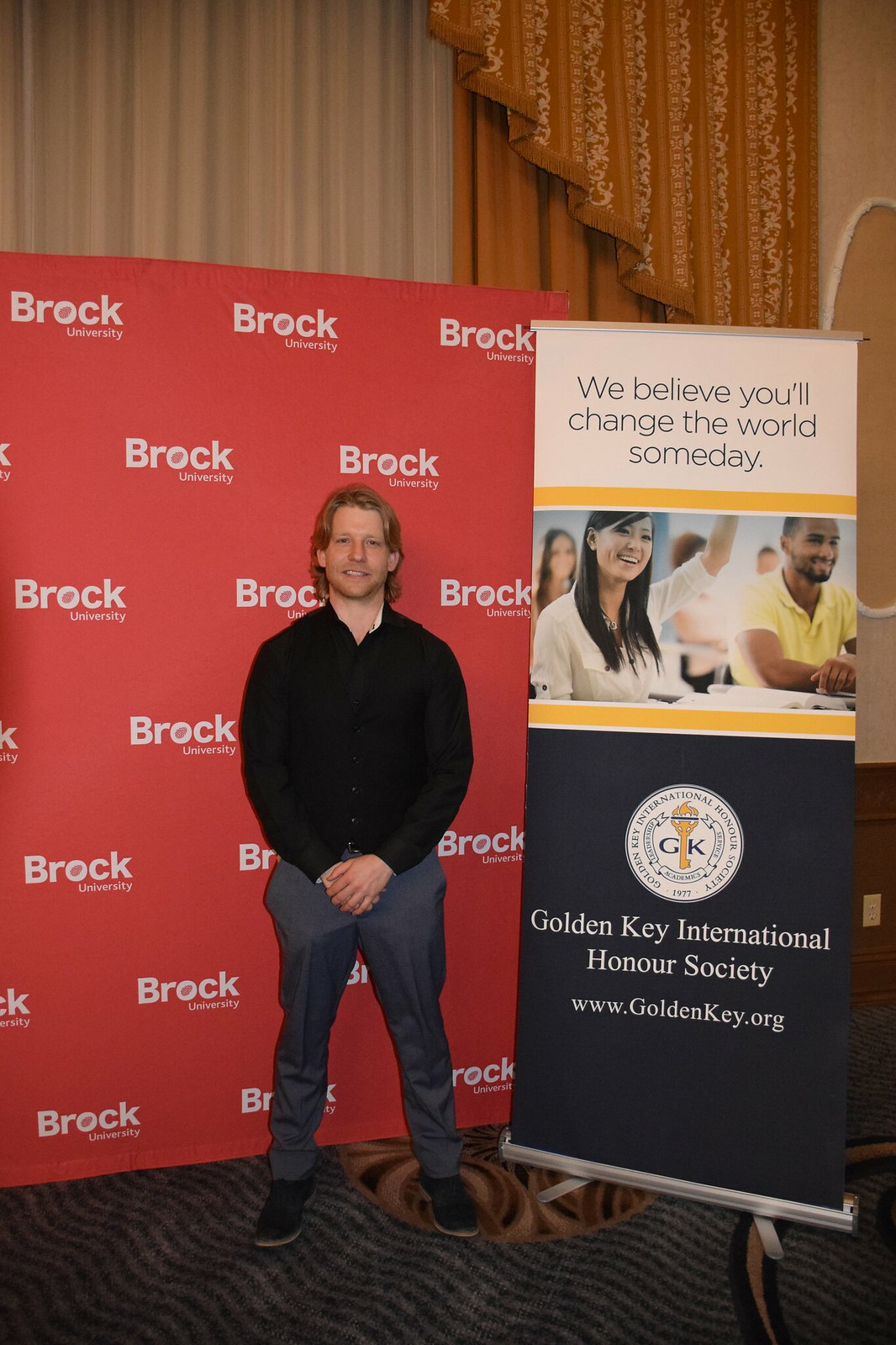The photograph captures a man standing in an expo area, positioned in front of a step-and-repeat banner adorned with the Brock University logo in white against a red background. To his right, there's a vertical billboard promoting the Golden Key International Honor Society. This billboard features a blue and white design with yellow trim and includes a headline that reads, "We believe you'll change the world someday," accompanied by an image of students in a classroom setting.

The man himself appears to be Caucasian, likely in his mid to late 20s or early 30s, with shoulder-length, brownish-blonde hair, and a somewhat awkward smile directed at the camera. He is dressed in a black shirt, blue or gray slacks, and dark shoes, possibly loafers. His attire is complemented by bracelets on his wrists, suggesting he might be a member of the Golden Key International Honor Society, as implied by the context of the banners surrounding him.